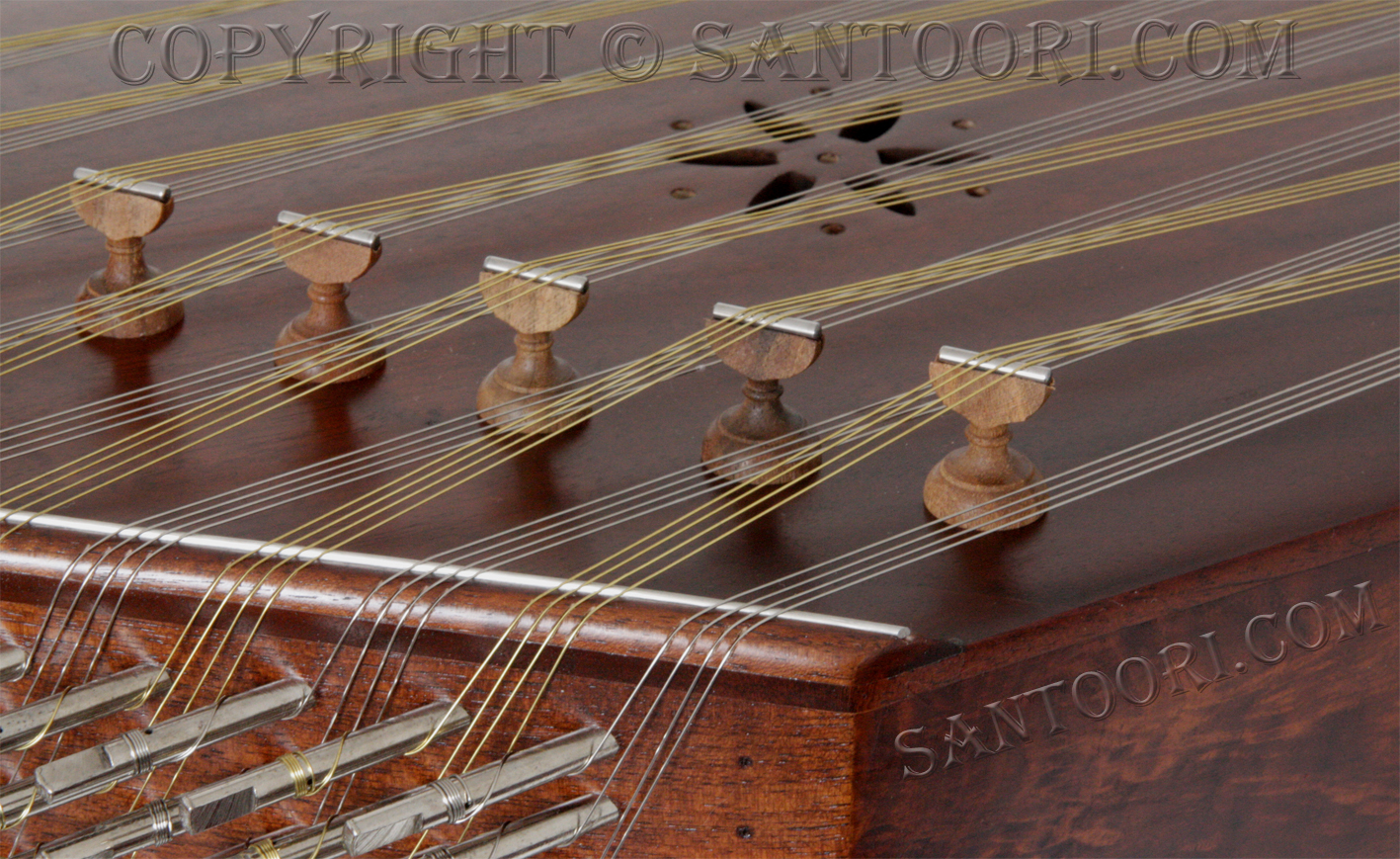This close-up photo captures a detailed view of a beautifully crafted stringed instrument. It features multiple groups of four to eight strings that are meticulously crossed over each other and stretch over a bridge. These strings are tethered to five wooden knobs, which have metal pieces on top, and are wound around long silver rods projecting from the end of the instrument, running back across its body. The instrument's design includes five frets and a flower-shaped carving in the center, accompanied by two small dots to the right of the metal rods. Prominently displayed on the instrument and within the image is the text "copyright santori.com" and "santori.com," indicating the possible make or brand of the instrument.